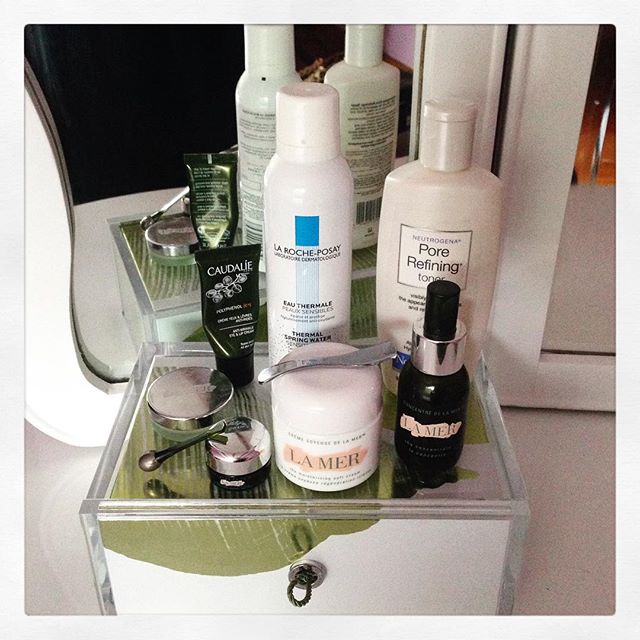This photo showcases a small, standalone storage container, likely made of clear plastic or glass. The container, viewed from an angled perspective, has a small lock on the front and is topped with an assortment of beauty products.

The items include a vintage Neutrogena Pore Refining Toner in a white, cream-colored bottle. In front sits a smaller black spray bottle labeled La Mer in thin black letters on a light pink logo strip, which also features a chrome cap.

Next to it, there is a closed cream jar also from La Mer, adorned with a similar pink and black label, possibly containing face cream. On top of this jar rests a silver beauty tool, whose function is unclear but might be for nails or clipping purposes.

To the left of these items are smaller containers with chrome or silver caps, though their labels are not discernible. Behind them is a small squeeze bottle from Caudalie, decorated with an image of grapes and other white text.

Dominating the center of the arrangement is a large La Roche-Posay bottle, marked with a distinctive blue rectangle and accompanying text, presumably containing thermal spring water. Reflected in a mirror with a white frame behind the container, the backs of these beauty products are visible, alongside another mirror to the right.

This setup, possibly part of a vanity, rests on a white surface with only a sliver of the surroundings on either side visible.